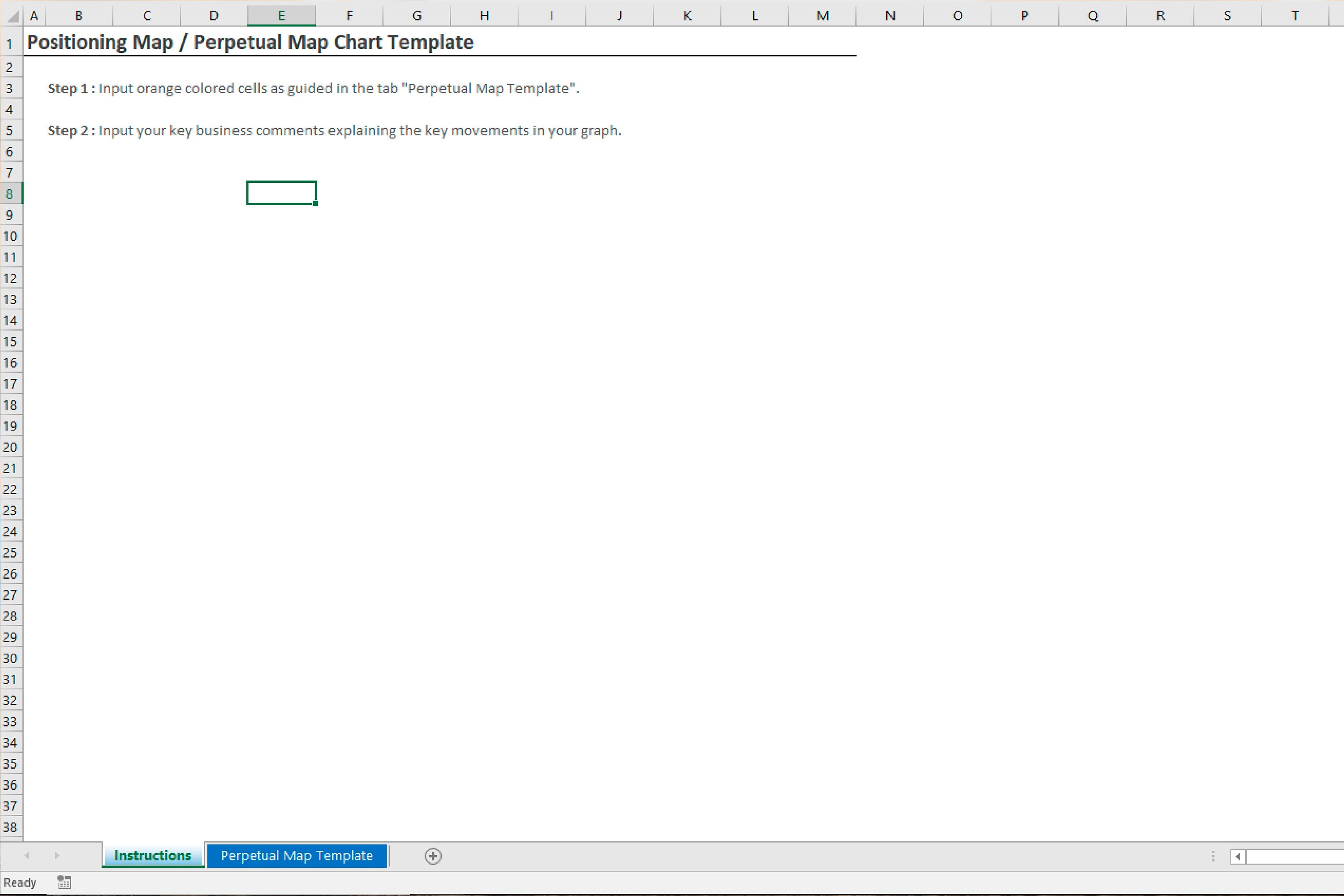The image displays a detailed view of a digital application with a predominantly white background and black text. At the top of the page, there is an interactive row of clickable letters from A to T that open corresponding tabs. Along the left side, there are numbered rows from 1 to 38. Both the letter "E" and the number "8" are highlighted and underlined in green, indicating they have been selected.

The title at the top of the page reads "Positioning Map / Perpetual Map Chart Template." Below this, there are two steps outlined: "Step one, input orange color cells as guided in the tab Perpetual Map Template," and "Step two, input your key business comments explaining the key movements in your graph." Additionally, at the bottom of the interface, the "Instructions" tab is highlighted in green, indicating it is currently active or selected.